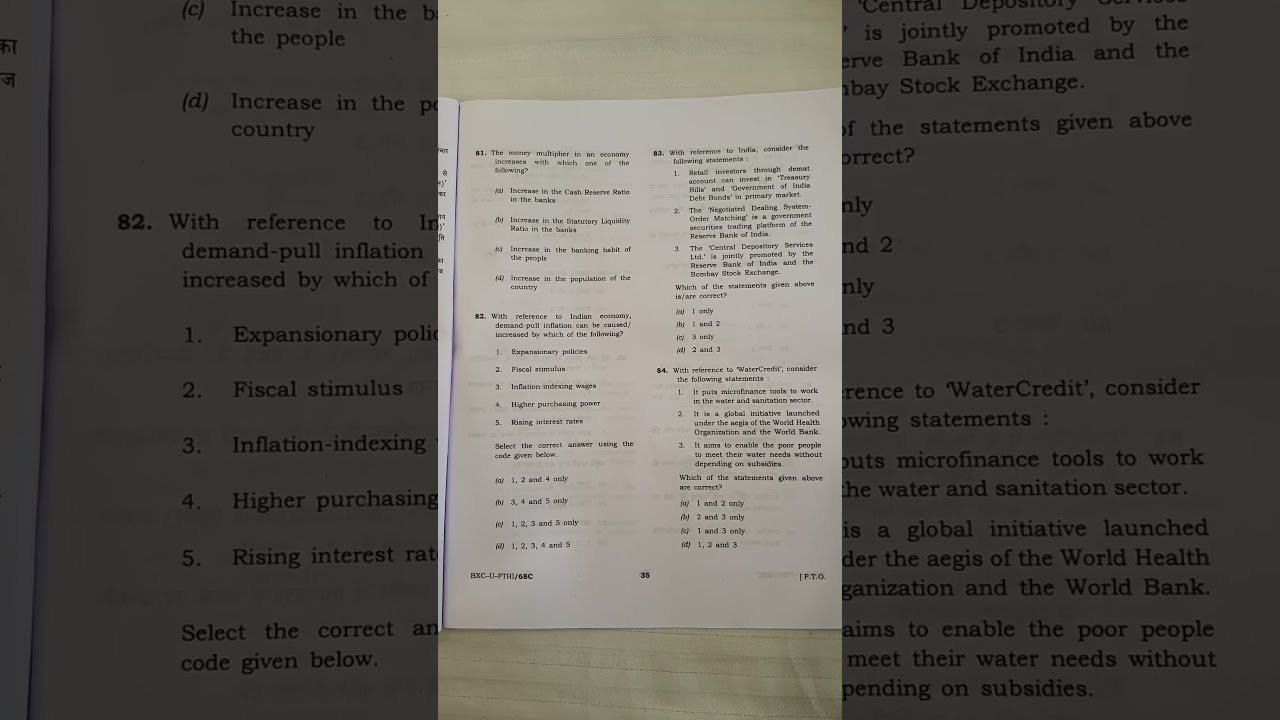The image shows a photograph of page 35 from a workbook or possibly a handbook, focused on economics topics. It features multiple-choice questions numbered 81 through 84. Question 81 discusses the money multiplier in an economy, asking which of several options can increase it. Question 82 relates to demand-pull inflation in the Indian economy, providing options labeled 1 through 5, with instructions to select the correct answer using a specific code. Question 83 involves considering statements about India and selecting the correct options from multiple choices. Similarly, Question 84 pertains to water credit, asking the reader to consider statements and choose the correct ones from the given options. The page is laid on a beige table, occupying most of the image, which appears slightly zoomed out, showing text such as "expansionary," "fiscal stimulus," "inflation indexing," "higher purchasing," and "rising interest." The overall setup gives the impression of a finance exam workbook in a clean, organized format.